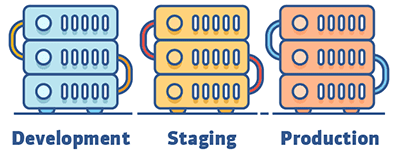The image features three rectangular robots that resemble speakers, each stacked one on top of the other. At the top of each rectangular section, there are five small circular openings, arranged in a row. From the topmost robot to the middle one, a blue hook is visible on the left side, and a similar blue hook connects the middle robot to the bottom one. Beneath the stack, there are two small circular stands supporting the robots.

The robots are color-coded as follows:
- The top robot is light blue with yellowish-orange handles.
- The middle robot is yellow with pink handles.
- The bottom robot is orange with blue handles.

Each robot has a label indicating its stage in a development process. The top robot is labeled "Development," the middle one "Staging," and the bottom one "Production."